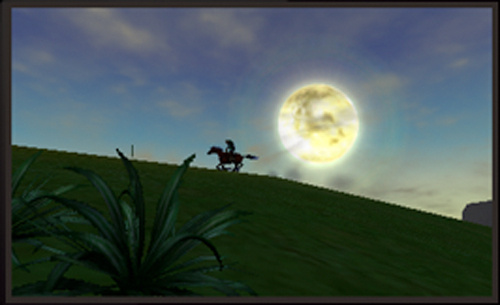In this captivating, computer-generated image, we see a dark, evening scene framed in black. The sky, still retaining its early evening blue hues, is dominated by a large, bright orb casting a golden glow—likely a full moon, given its size and luminosity. Gray and white clouds drift across the moon, adding depth and texture to the sky.

In the foreground, a lush green hill stretches across the scene. Prominent on this hill is a silhouette of a person on a galloping horse, their outlines starkly black against the illuminated sky. The horse's tail streams back, suggesting the speed and urgency of their movement as they head towards the left side of the frame.

Closer to the bottom left corner of the image, detailed green plants with long, elegant leaves add to the sense of depth and realism in the scene. Despite the pixelated texture, the elements of the image create a vivid and dynamic depiction of a moonlit landscape, with the rider and horse racing through the night.